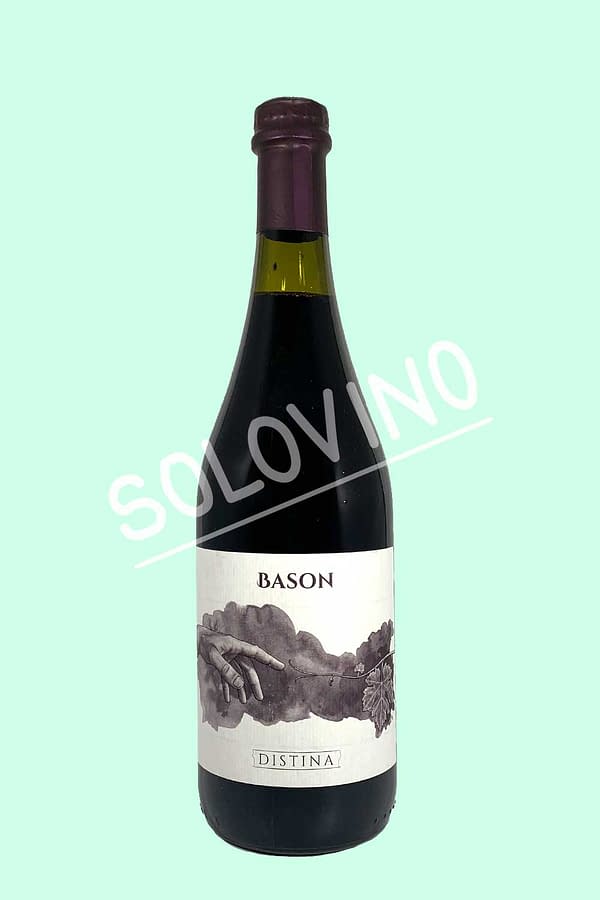The image is a graphic advertisement prominently featuring a sealed, dark-colored bottle of wine with a tall neck, set against a seafoam green background. The bottle is adorned with a white label that reads "BASON" at the top and "DISTINA" underneath. The label also features a black and white drawing reminiscent of Michelangelo's Sistine Chapel, depicting a hand reaching out towards a grapevine. Diagonally across the bottle, in white text, is the word "SOLOVINO," adding a dynamic element to the composition. The image is minimalistic yet detailed, with a focus on the elegant presentation of the wine bottle and its artistic label.